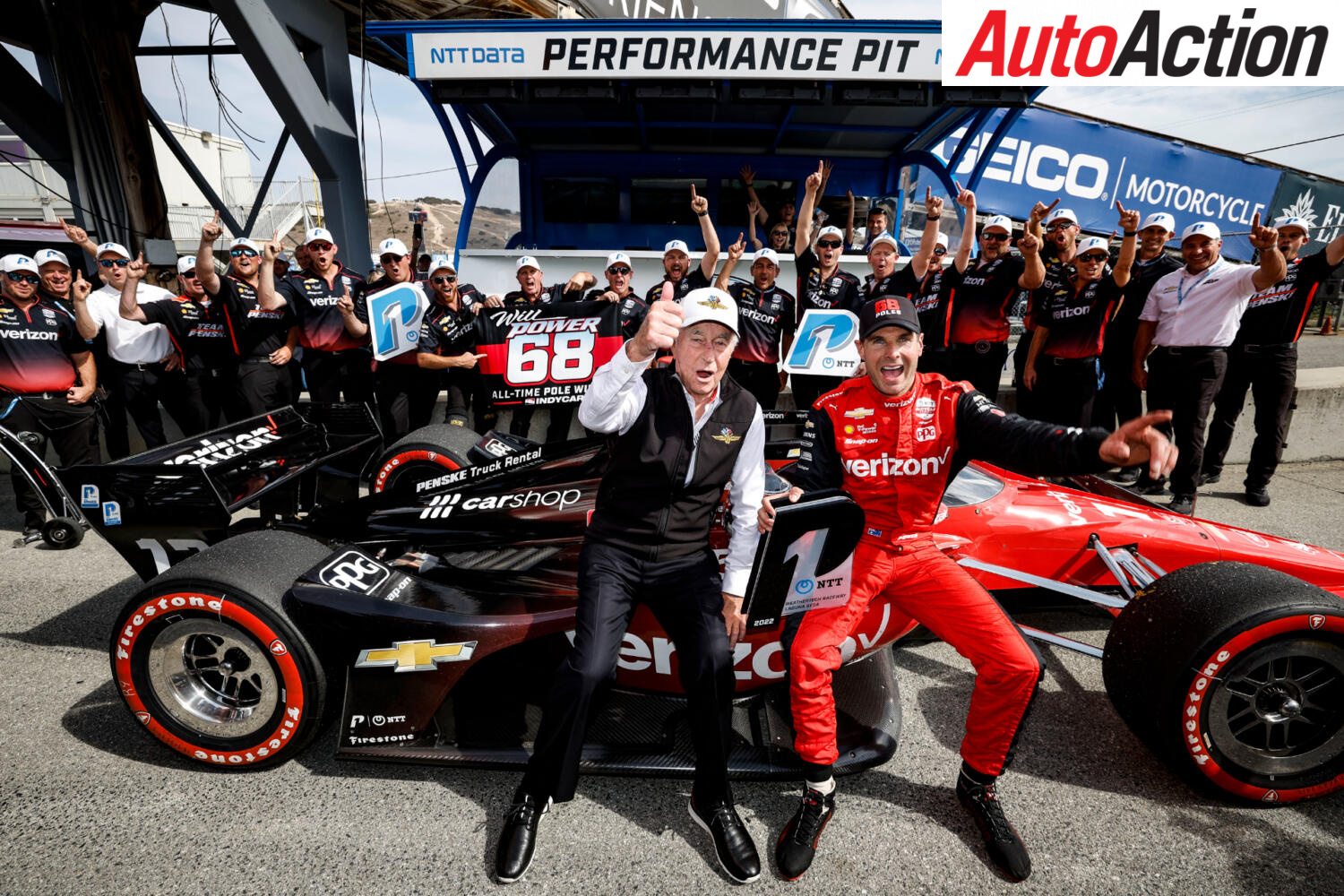In this vivid and energetic scene from a modern NASCAR event, the image showcases a dynamic celebration at the NTT Data Performance Pit. Prominently featured in the foreground is a sleek red race car adorned with black wheels trimmed in red and emblazoned with myriad sponsor logos, including Verizon, Firestone, Penske Truck Rental, and PPG. Perched atop the car is a jubilant, presumably victorious driver in a distinctive red and black suit with Verizon branding, complete with a coordinating cap and black shoes. 

Next to the driver, an older gentleman, likely the team owner, is dressed in a white button-up shirt, black vest, black pants, and a white hat. He enthusiastically gives a thumbs-up to the camera, embodying the celebratory spirit of the moment. 

The backdrop is a lively tableau of fans and crew members, their excitement palpable. They wave their arms, signaling 'number one' and brandishing signs like "Willpower 68" and "P1," all under the bright, sunny sky. Many of them sport white hats and some are in black and red Verizon-branded shirts, contributing to the unified team identity. 

Overall, this detailed depiction captures the triumph and euphoria of car racing at its finest, set against the bustling atmosphere of a high-stakes NASCAR race.